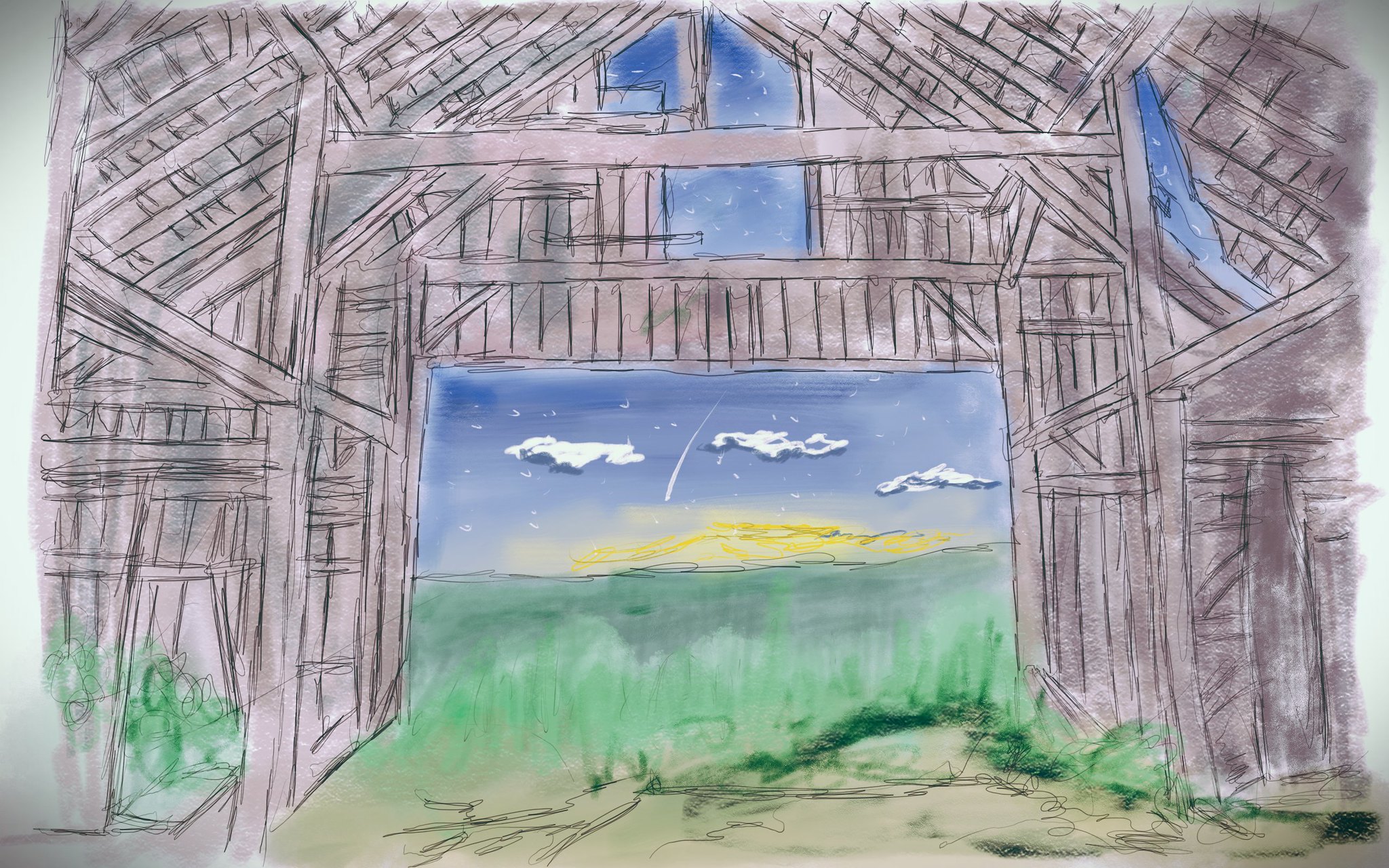This detailed drawing, rendered on a rectangular sheet of paper in landscape orientation, features a rustic barn open to the outdoors. The barn, depicted with a light brown structure, appears somewhat dilapidated, with visible holes near the ceiling area. In the background, a light green grassy field stretches out under a dark blue sky, punctuated by three distinct clouds. Through the barn's opening, a partial view of a dusky sunset unfolds, showcasing a vibrant yellow sun beginning to disappear beneath the horizon.